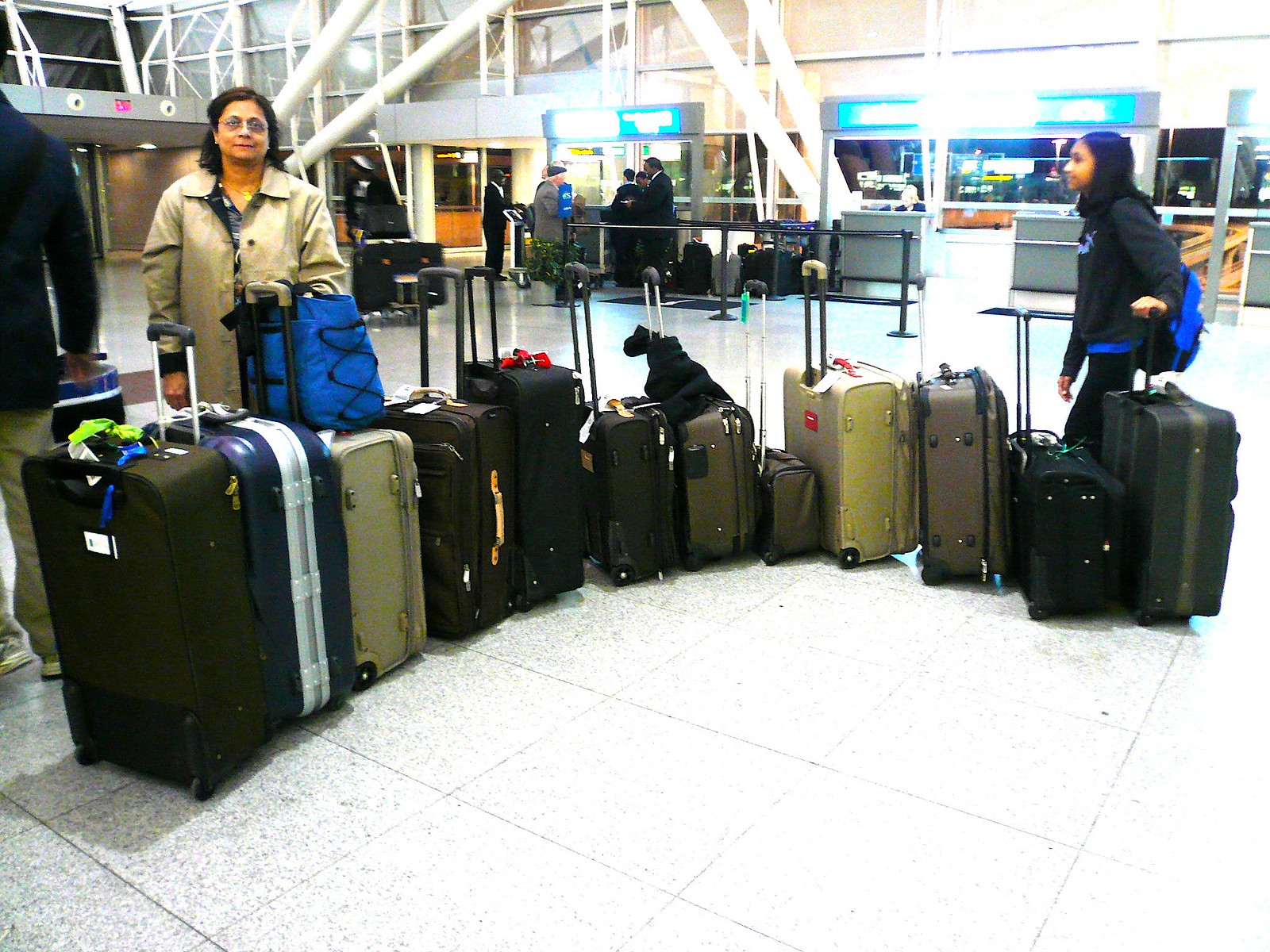In this detailed airport scene, an older woman with long black hair, wearing glasses, and dressed in a khaki-overcoat, stands prominently in the foreground against a white-gray speckled tile floor. She is holding a blue bag on her left arm and stands beside an array of 14 suitcases of varying sizes and colors, meticulously arranged in a semi-circular fashion from left to right. The luggage includes black, brown, and gray carry-ons, each with retractable handles and wheels.

To the right of the woman, a younger brown-skinned girl with shoulder-length hair, wearing a dark blue sweatshirt and a matching blue book bag, stands looking towards the older woman. Her left arm extends over the suitcases, adding to the sense of interaction between the two.

In the background, there is a bustling check-in area adorned with blue-lit signs above the counter windows, which are busy with travelers gathering their luggage. Visible overhead are pipes running along the ceiling, adding to the industrial ambiance of the airport.